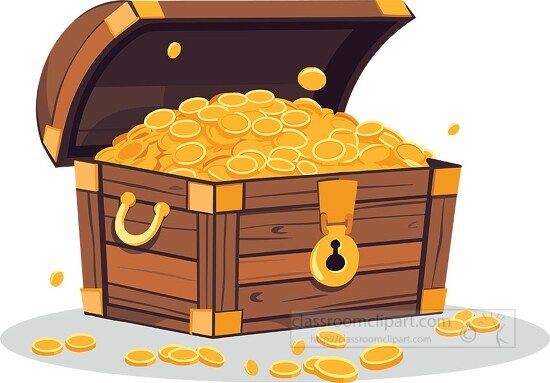The horizontal, rectangular illustration features a classic pirate-style wooden treasure chest prominently in the center, with its bottom left corner facing the viewer. Adorned with gold handles on the sides and reinforced with gold brackets at the corners, the chest is detailed with a circular lock on the front. The lid, made of brown wood with a barrel-shaped top, is open to reveal a mound of gold coins inside. These coins, varying in shades of gold, with some resembling orange slices with darker centers and lighter rims, overflow from the chest. Several coins appear to be mid-air, suggesting movement as they spill out, with quite a few scattered on the ground around the chest. A light gray, oval-shaped shadow is cast in front of the chest. The illustration includes a subtle gray watermark in the bottom right corner that reads "classroomclipart.com," indicating it is a color illustration clipart.